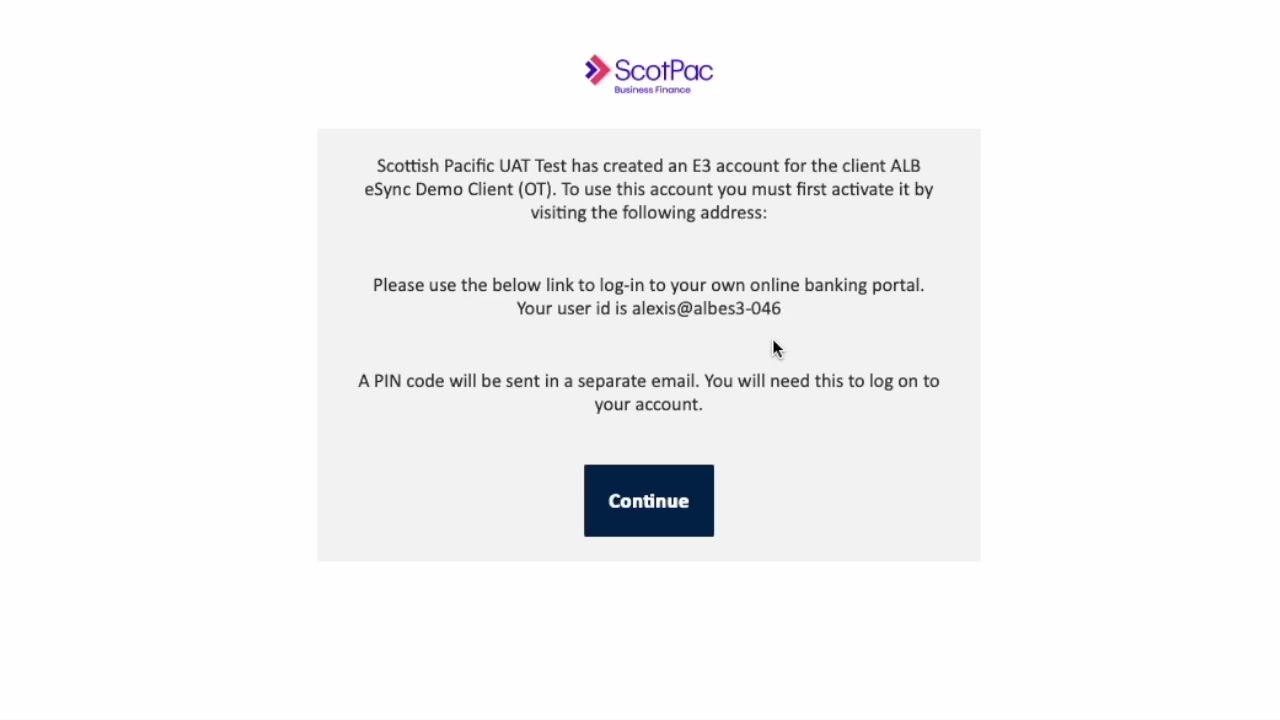This image is a screenshot from a website interface. It features a clean white background with a prominent box in the center. At the top of the interface, there is a white header section displaying an icon and the name "Scott Pack" in purple font with the letters "TS&P" capitalized, indicating a focus on Business Finance. Below the name, there is a logo featuring two arrows pointing to the right: a smaller purple arrow on the left, encompassed by a larger pink arrow.

Beneath the header, there is a gray, landscape-oriented box containing informative black text. The text announces that "Scottish Pacific UAT Test" has created an E3 account for the client named "ALB E-Sync Demo Client OT." The message instructs the user to activate the account by visiting a specified address and to log into their online banking portal using the user ID "alexis" at "alpes3-046." It notes that a separate email will be sent containing a PIN code necessary for account login.

At the bottom of the gray box, there is a blue, rectangular button with white font, labeled "Continue," suggesting that accessing this button would lead the user to the next step in the login or account activation process.